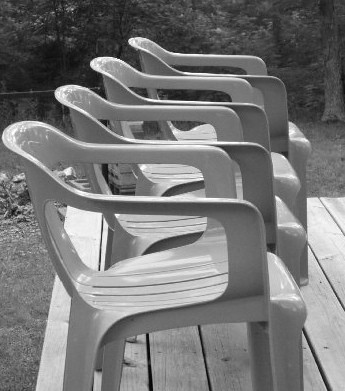This black-and-white photograph captures a serene backyard scene featuring a row of four plastic patio chairs on a light-colored wooden deck. The deck, composed of vertical wooden planks, lacks a railing and is set against a backdrop of trees, suggesting a yard with abundant greenery and possibly a chain link fence. The chairs, facing to the right and slightly misaligned from each other, are of a common, inexpensive type typically used outdoors and possibly stackable. Each chair has comfortable armrests, a bowed backrest, and slats in the seats to allow rain to pass through. The light-colored wood of the deck contrasts with the shades of gray in the grass and foliage around it, showcasing the simplicity and tranquility of the outdoor setting.